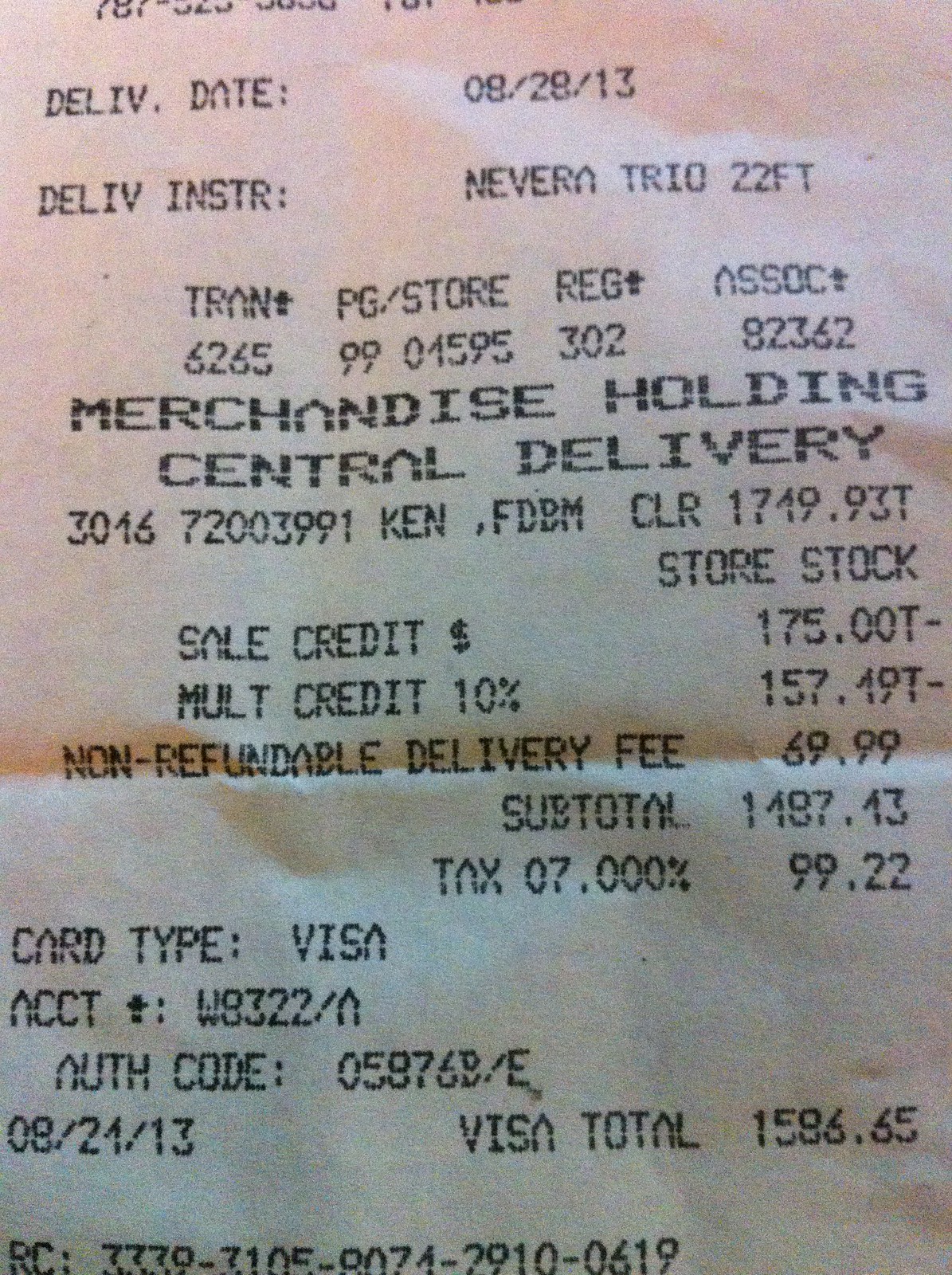Receipt detailing a delivery order

Delivery Date: August 28, 2013

Delivery Instructions: 
- Item: Nivera Trio, measuring 22 feet 

Transaction Information:
- Store: Trans PG Store
- Registration Association: 62659901595
- Registry: 302 Association 82362
- Merchandise Holding: Central Delivery (displayed in larger, bolder text)

Purchase Details:
- Product Code: 3-30-16-7-2-2-7-2-0-0-3-9-9-1 Ken
- Description: FDBM Clear CLR
- Item Price: $1,719.93 
- Store Stock Sale Credit: Cash refund of $175.00 
- Multi-Credit Discount: 10%, amounting to $157.49 
- Non-refundable Delivery Fee: $69.99 
- Subtotal: $1,487.13 
- Tax (7%): $99.22 

Payment Summary:
- Card Type: Visa
- Account Number: W832NN-A
- Authorization Code: 05876B-E
- Transaction Date: August 21, 2013
- Visa Total: $1,586.85 
- Reference Number: 3339310580742910619